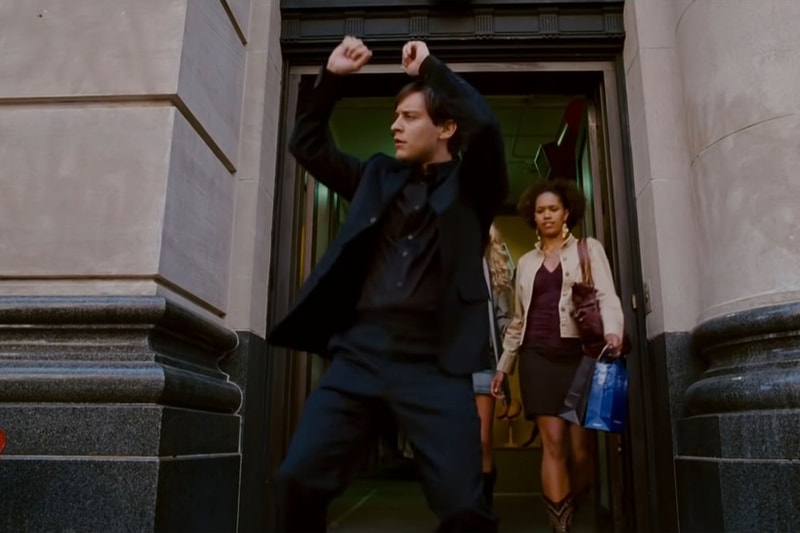In this image from the movie "Spider-Man," Tobey Maguire, portraying Spider-Man, is exiting a two-tone stone building with light columns and a dark base, possibly obsidian or viridian in color. He is dressed in a casual black suit with a button-down shirt, no tie or bow tie, and dark pants, potentially jeans, and is exuberantly dancing with his arms raised and fists in the air. Following him out of the building are two women. One is African American, wearing a dark-colored skirt, a burgundy v-neck shirt, a tan jacket, and carrying two shopping bags in addition to a burgundy purse. The other is a blonde dressed in a dark blue shirt and a denim skirt, partially visible. The jubilant atmosphere suggests Tobey's character is quite happy, although the reason for his excitement remains unknown.